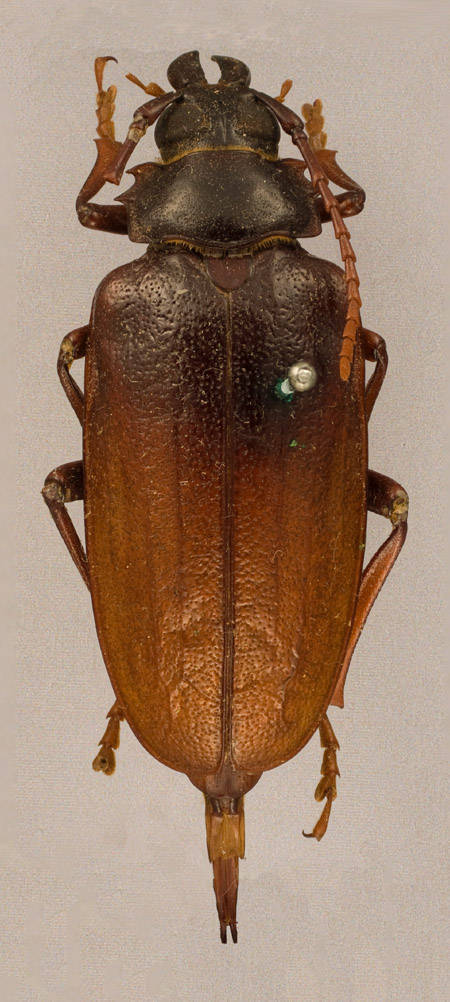This close-up image captures a highly detailed view of a single insect, appearing to be a dead cockroach, centered perfectly against a light tan background that fades to a lighter shade towards the bottom. The insect's most prominent features include its black head with two protruding horn-like structures, and a distinctly dark brown line running down the center of its rounded rectangular body. The body itself exhibits a color gradient from darker brown at the top, transitioning to a lighter brown. Notably, there is also a subtle touch of green on the shell. The cockroach's anatomical details are thoroughly visible, including its thin, dark brown legs that fade to a lighter brown, with two legs near the head and two on each side, all tucked close to its body. A tail-like appendage extends from the rear. The photograph displays no text, and the insect's meticulous presentation suggests it could be of interest to someone researching or fascinated by bugs.